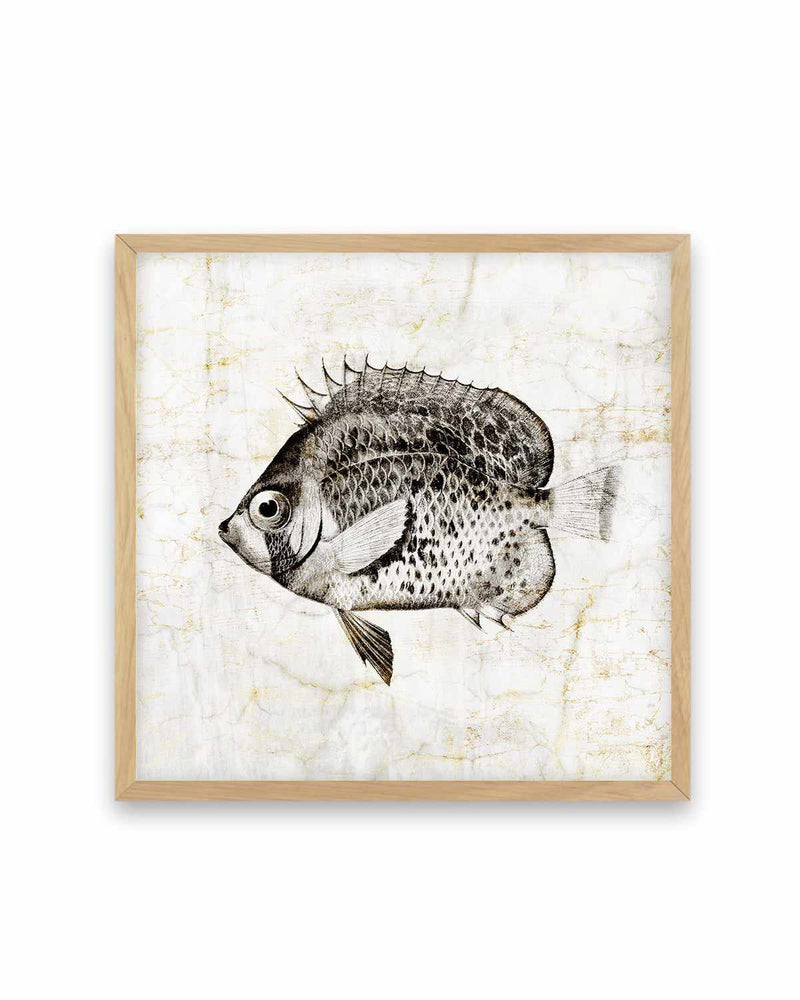This image showcases a highly detailed framed print of a fish with a light, thin wooden frame that encloses the artwork. The central focus of the image is a meticulously sketched fish, executed in black colored pencils or charcoal. The background is predominantly white with varying textures of brown, lending a subtle depth to the composition. The fish is swimming to the left, featuring a pronounced eye with a distinct pupil. Its body is short and broad, adorned with an intricate pattern of black and white scales that transition smoothly from dark to light. The fish has small, short fins and a petite tail, with a spiky dorsal fin adding to its dynamic appearance. The overall lack of bright colors emphasizes the monochromatic artistry, reinforcing the detailed texture of the fish against the simple background.